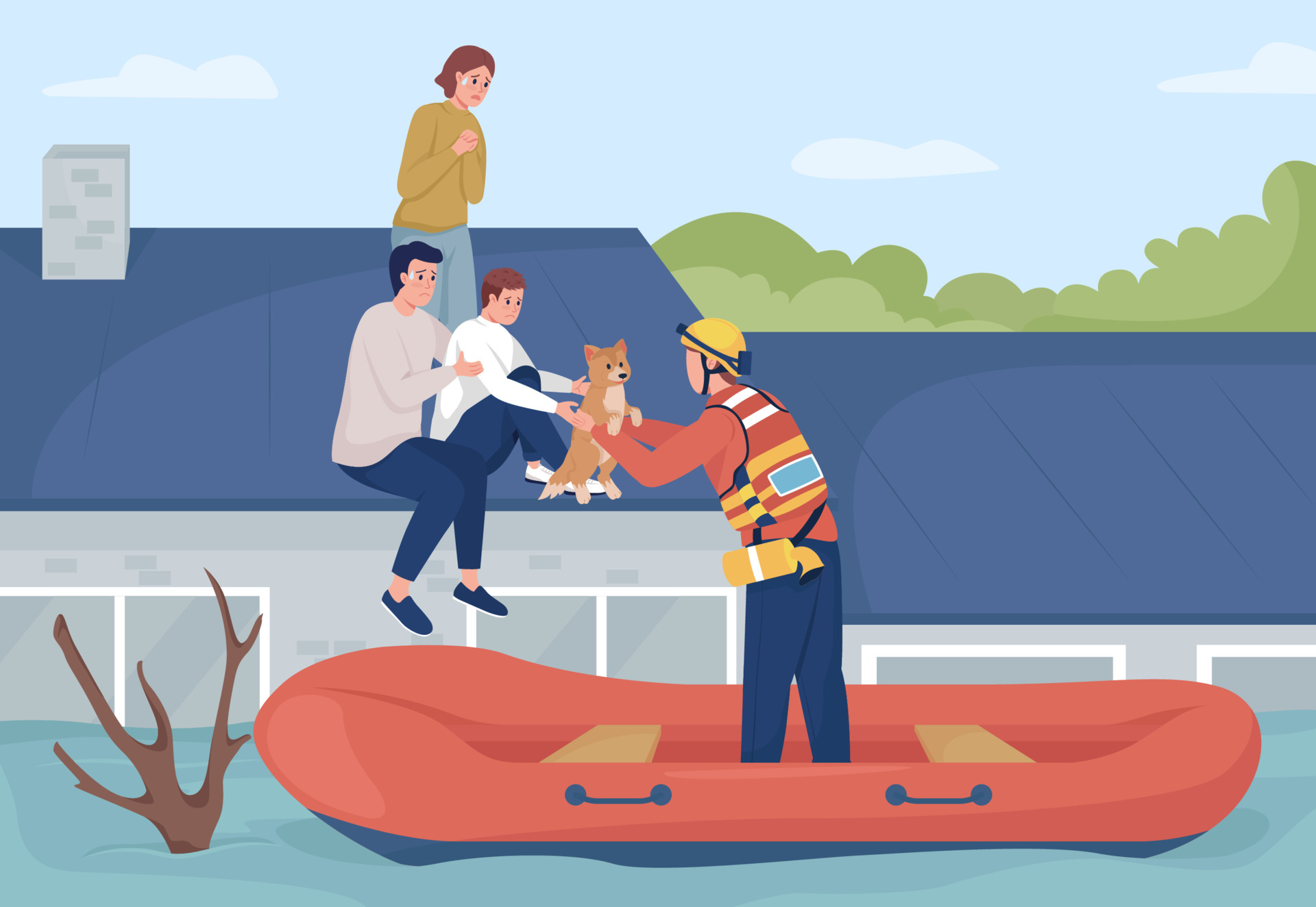This detailed color illustration depicts a dramatic rescue scene set in the aftermath of a flood. A family consisting of a woman, man, and a child along with their dog are stranded on the slanted roof of a gray-brick house with water levels rising above the windows. The roof, colored blue, features a prominent gray brick chimney. 

The family's distress is palpable as they stand on the roof: the woman, with light brown hair, is dressed in a green sweater and blue pants, folding her hands with a tear running down her face. The man, donning a gray sweater and blue pants with blue shoes, has deep blue hair and an anxious expression. The child, wearing a white sweater, blue pants, and white shoes, is handing their light brown, fox-like dog to the emergency worker.

The rescue worker, positioned in an orange inflatable raft with a blue underbody, wooden seats, and blue handles, is the central figure of the scene. Equipped with a yellow hard hat adorned with a blue light, an orange safety vest lined with yellow stripes over a long-sleeved orange shirt, and blue jeans, he reaches out to receive the dog from the child. The backdrop presents a serene, albeit stark contrast to the urgent situation, featuring blue skies with white clouds and green leafy trees.

In the foreground, a tree branch sticks out of the floodwater, further emphasizing the height of the rising water around the house. This visually compelling illustration vividly captures the desperation and hope amidst a crisis, emphasizing the coordinated efforts of the rescue mission.